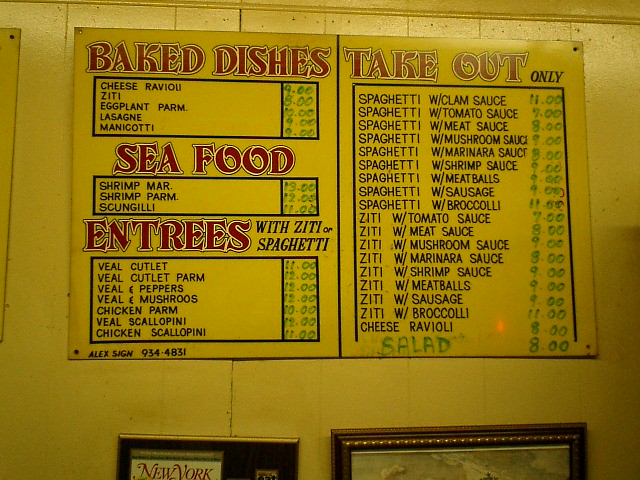Here's a refined and detailed caption:

"The image showcases a vibrant yellow wooden wall adorned with an expansive menu divided into three distinct sections, each highlighted by bold red and black lettering. At the top, there are two framed pictures with ornate gold frames. Directly above them, a large dual-sided yellow sign catches the eye.

The left section of the sign details "Baked Dishes" in prominent red letters, followed by a black panel listing an array of options: Cheese Ravioli, Ziti, Eggplant Parm, Lasagna, and Manicotti. Further down, "Seafood" is highlighted in red, beneath which a black panel lists dishes such as Shrimp Marinara, Shrimp Parmesan, and Scungilli.

The middle section titled "Entrees" in red letters offers a variety of dishes served with ziti or spaghetti. The black panel elaborates on choices like Veal Cutlet, Veal Cutlet Parmesan, Veal and Peppers, Veal and Mushrooms, Chicken Parmesan, Veal Scallopini, and Chicken Scallopini.

The right section is headed by "Take Out" in striking red letters. The black panel underneath features an extensive list of pasta dishes: Spaghetti with various sauces (clam, tomato, meat, mushroom, marinara, shrimp), Meatballs, Sausage, Broccoli, and Cheese Ravioli. The menu also includes Ziti variations with similar sauces and toppings. At the very bottom, "Salad" is written in green letters, rounding out the extensive menu offerings."